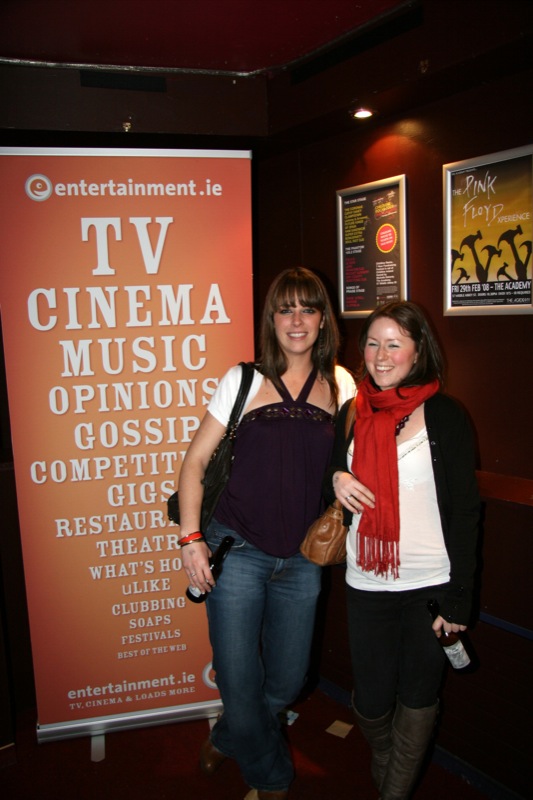The image captures two young women posing in front of a tall, orange banner with white text that reads "entertainment.ie, TV, cinema, music, opinions, gossip, competitions, gigs, restaurants, theaters, what's hot, clubbing, soaps, festivals." Both women, who have shoulder-length brown hair and light complexions, are smiling and holding beer bottles. The woman on the right is wearing a white blouse, black pants, tall brown boots, a red scarf, and a long black cardigan. She also has a light brown purse slung across her body and features notably rosy cheeks. The woman on the left is dressed in a black top over a white shirt, blue jeans, and carries a black purse on her left shoulder. Without any accessories, she complements the stylish look of her companion. Behind them, the setting is dimly lit with visible silver-framed posters, including one for "The Pink Floyd Experience." The banner they stand in front of indicates that the location is associated with an entertainment website offering various options in TV, cinema, music, and more.